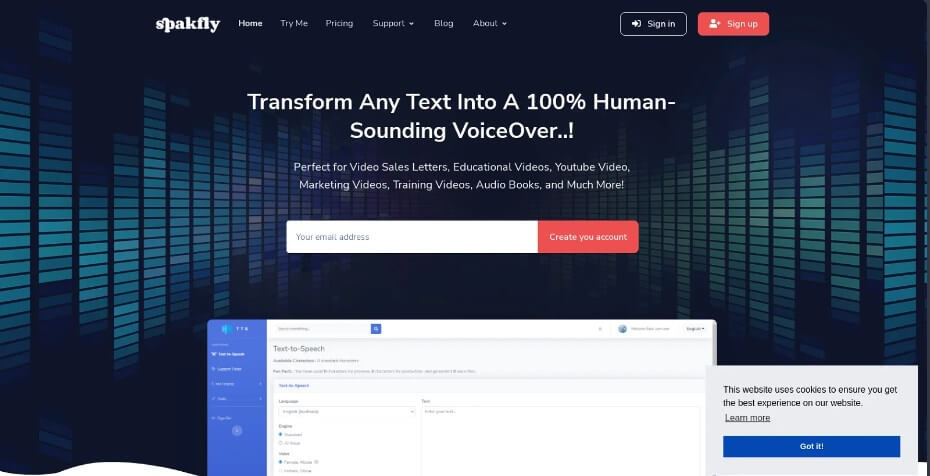The screenshot appears to capture a section of a website designed with a dark, nearly black, background. On the left and right edges of the screen, there are small blue rectangles resembling old-style equalizer bars that move up and down in varying heights. 

At the top portion of the page, somewhat left of center, the text "SPAC Fly" is prominently displayed in large white font. Adjacent to this title are navigation options in a smaller font: "Home," "Try Me," and four other menu items with drop-down capabilities, though these are somewhat difficult to read due to their small size.

Towards the top-right section, there are two buttons: "Sign In" with a dark background and "Sign Up" highlighted in red.

Below this header, centrally located, is a headline in white text stating: "Test trend – Transform any text to a 100% human-sounding voiceover!" 

Under this headline are two rows of text positioned centrally. Following these text rows, there is a white input box with a red button attached to the right side, suggesting a space where users can type in their own text.

Towards the bottom of the screenshot, a part of the website product showcase becomes visible, with the left section in blue and the right in white. At the bottom left corner, a subtle gray notification window informs users that "This website uses cookies to ensure you get the best experience," accompanied by a blue "Got it" button.